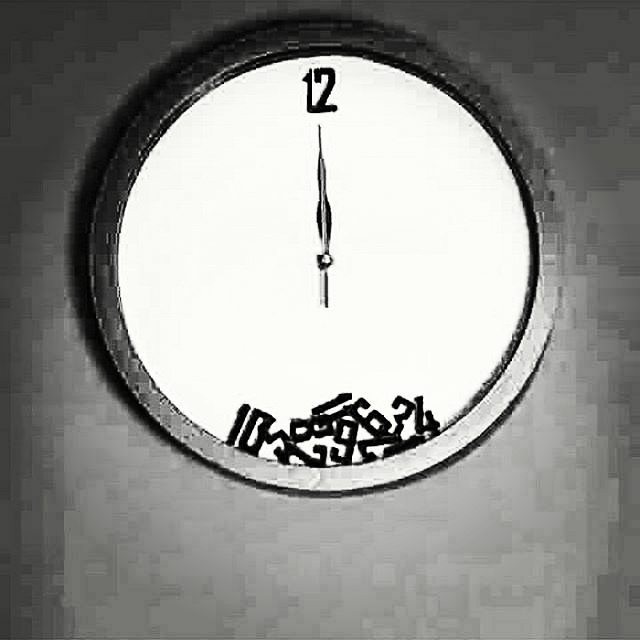In this pixelated image, a round clock hangs on a wall, displaying an intriguing and unconventional design. The clock features a distinctive baffled frame that draws attention to its artistic form. The clock face is stark white, creating a sharp contrast with the dark accents of the hands and numbers. Singularly striking, the clock has only one hand, a sleek indicator pointing directly upward to the number 12, which is the sole number in its correct position. Adding to its unusual charm, the bottom of the clock face showcases a chaotic pile of the remaining clock numbers, as if they have tumbled from their standard positions, creating a heap of numerals haphazardly stacked together. The visual effect captivates the viewer, blending traditional timekeeping with a playful element of disarray.